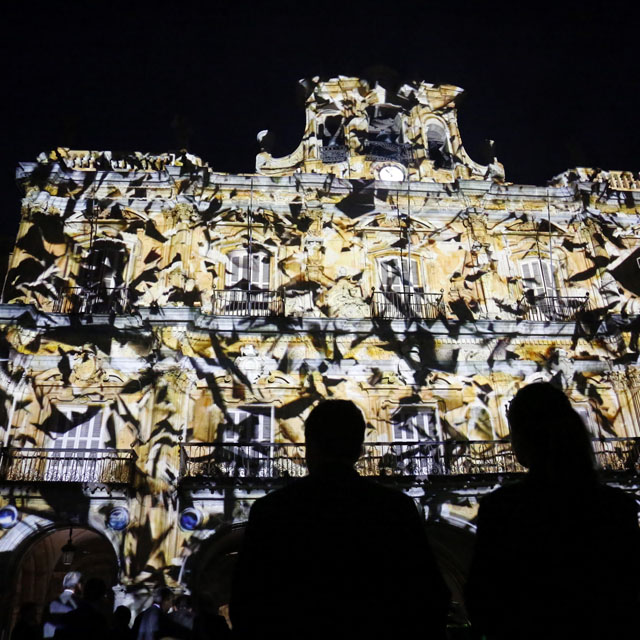This image, square in shape, captures a nighttime outdoor scene dominated by a very large, possibly colonial Spanish-style building that stands about three stories high. It's an impressive structure with distinct architectural features such as black gated balconies and white-trimmed windows, and it notably has a house-like section positioned towards the middle right of the frame. The building’s façade is bathed in shadows, adding to its dramatic appearance, while a captivating and intricate light show casts a unique, funky pattern across its surface. At the very top, a large clock is faintly visible, blending into the darker tones. Below, at the bottom right of the image, two people are silhouetted against the darkness, appearing almost blacked out, as they stand near a brown door with gray or silver handles. The entire scene is devoid of any text and is focused on the visual interplay between the light patterns on the building and the deep shadows that cloak the scene. Additionally, there seems to be a scattering of birds or similar shapes in the sky, contributing to the mysterious ambiance.